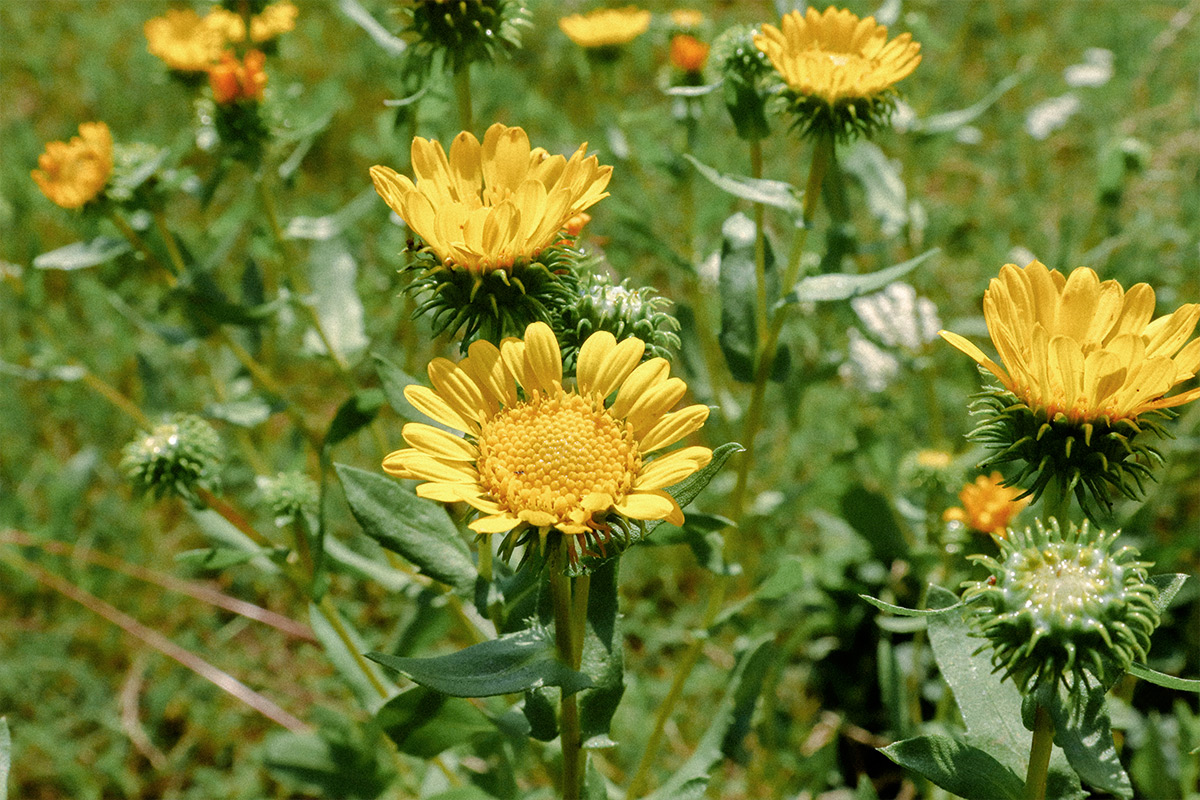This vibrant photograph captures a picturesque scene of wildflowers in a grassy field, with a particular focus on clusters of bright yellow flowers set against a backdrop of lush green leaves and stems. The yellow petals and green parts of these flowers resemble sunflowers or possibly gumweed, though a few are adorned with small dots on their centers. The image prominently features various stages of bloom: some flowers are in full bloom with vivid yellow petals, others are partially open, and some have lost their petals entirely, displaying bare centers with surrounding green spikes. Interspersed among the yellow blossoms are a few orange flowers, adding a contrasting burst of color to the scene. The overall array of delicate flowers, some fully open and others either budding or decayed, makes for a vivid and detailed composition of nature's cyclical beauty.